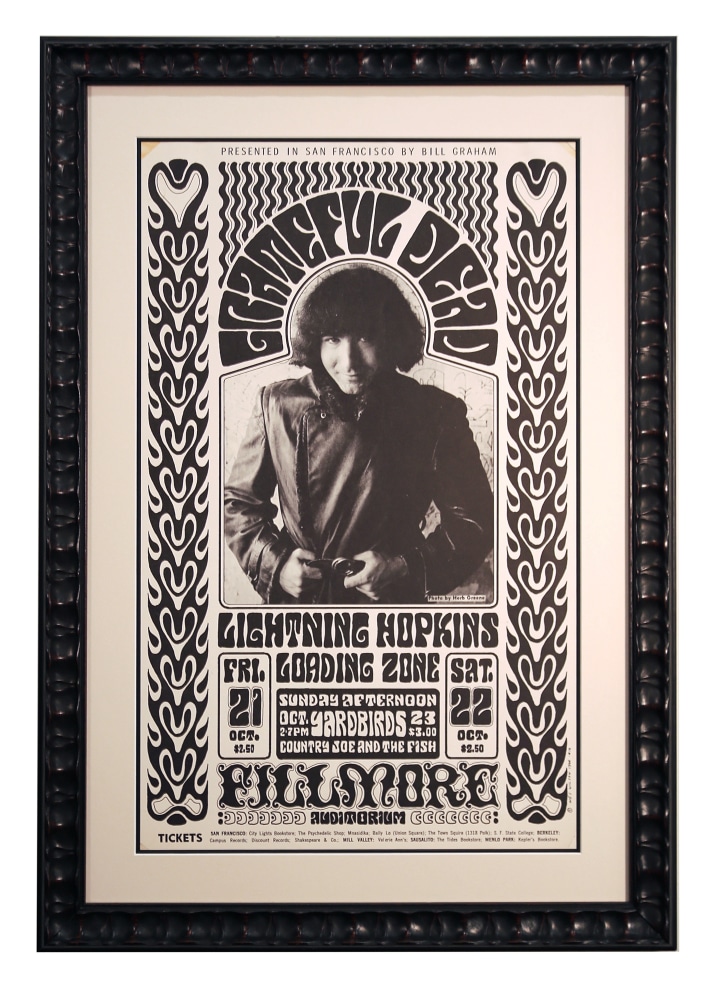The image showcases a vintage black-and-white rock-and-roll poster framed in an ornate, dark wood frame with numerous engravings. This product is likely intended for commercial listings or catalog photos, given its edited background that creates the illusion of the frame floating in a white void, emphasizing the product itself. The frame isn't just plain; it features various indents and ridges, enhancing its decorative appeal. The poster, set against a light cream or beige background, centers on a photograph of Lightning Hopkins wearing a black coat with a side zipper. He has long, curly black hair and is pictured from his head to his mid-waist, with his hands grasping his belt. Surrounding his image is black text, detailing a concert presented in San Francisco by Bill Graham. The poster highlights the dates "Friday, 21st October, $2.50" and "Saturday, 22nd October, $2.50." Additional artistic elements include a vertical decorative banner with heart shapes and the names of other acts. Most notably, the names "Lightning Hopkins," "Loading Zone," and "Fillmore Auditorium" appear in black decorative fonts, creating a striking and nostalgic piece of vintage poster art.